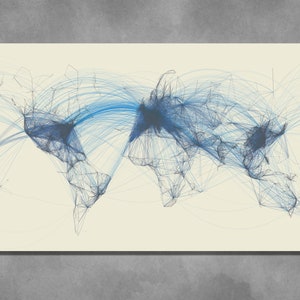This square image features a textured gray border at the top and bottom, resembling concrete, framing a white central canvas. The focal point is an abstract representation of a world map, primarily illustrated with shades of blue and black. The blue and black lines, varying in width and direction, form an intricate web that suggests air travel routes. On the left side, the shapes of North and South America are discernible, transitioning through Africa and Europe centrally, extending to Asia and Australia on the right. The dense clustering of lines signifies major flight paths, particularly highlighting the northeastern United States, Europe, and South Asia, while sparser lines stretch towards less populated regions such as Alaska and the southern tip of South America. The overall visual effect is an abstract yet evocative depiction of global connectivity.